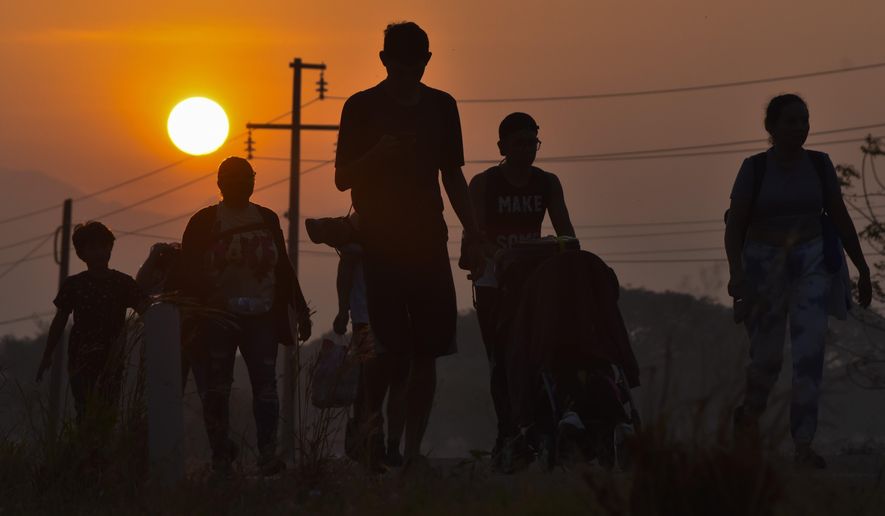The photograph depicts a group of six silhouetted individuals walking along a road at sunset. The vibrant orange sky dominates the upper half of the image, with the bright sun positioned in the upper left corner, transitioning into a purple-hued horizon. From left to right, the figures are staggered and vary in height and activity. The far-left figure, possibly a child, holds an upright stick or rifle. Beside them is a taller figure, seemingly unencumbered. The central and tallest silhouette, appearing least burdened, possibly masks part of a sixth person. To the right of center, another figure maneuvers a wheelbarrow-like object laden with baggage. The far-right silhouette, identified by acid-washed blue jeans, appears to be female. All figures are rendered in dark shadow, offering minimal detail due to the intense backlighting of the setting sun, creating a dramatic visual contrast against the vivid sky.